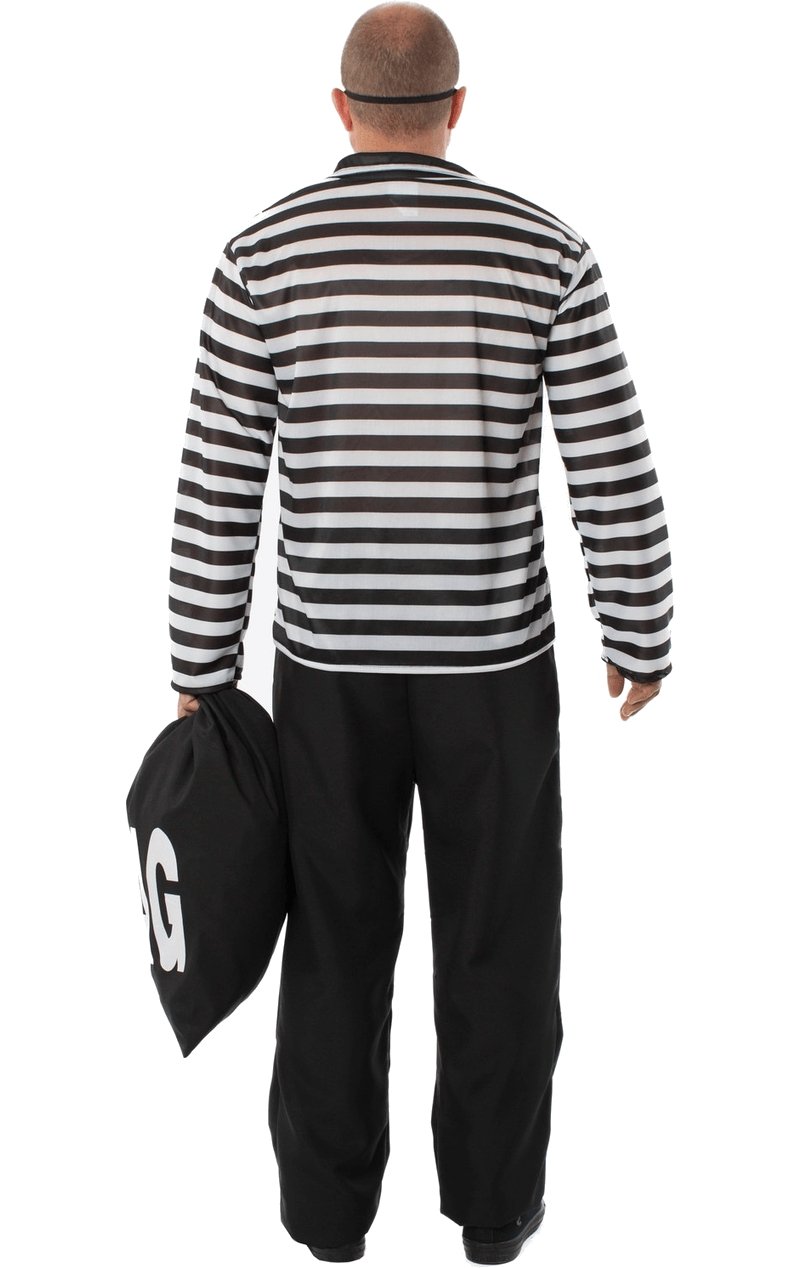A man is standing facing away from the viewer against a clear, white background. He has a sandy blonde, closely shaved head with a noticeable bald spot on top, and a skinny black band wraps around the back of his head just above his ears, resembling a mask strap. He is wearing a long-sleeved shirt with horizontal black and white stripes and a black collar. His outfit includes baggy black pants and black shoes, the back heels of which are visible. He is holding a black cloth bag with a drawstring in his left hand, which prominently features a large, white capital letter "G." His arms are slightly extended out to his sides, creating a small gap between them and his body.